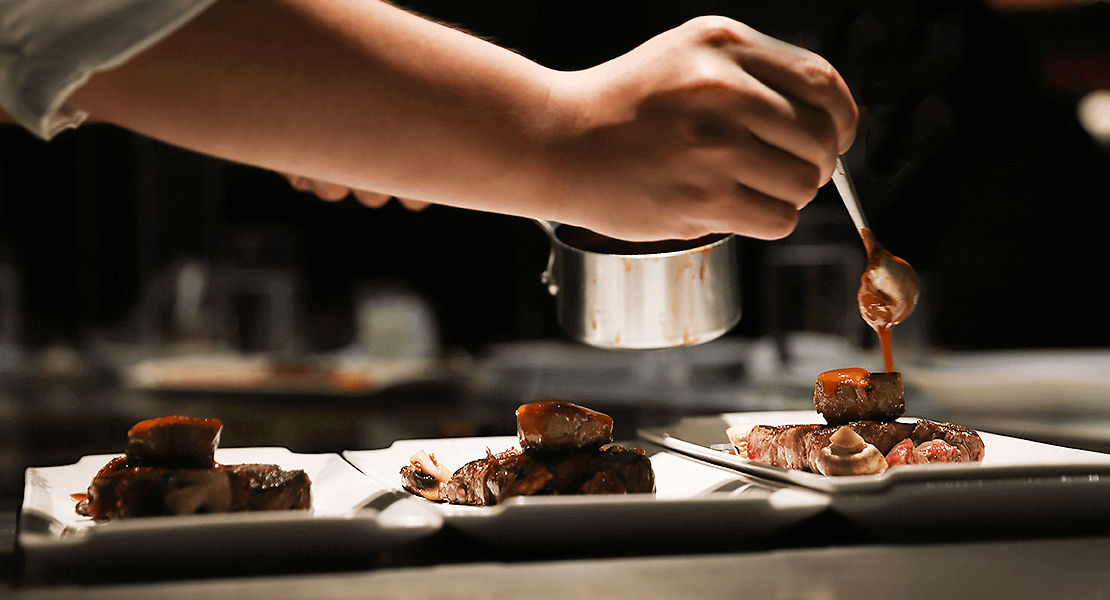The photograph captures a meticulously crafted kitchen scene focused on a fine dining food presentation. In the foreground, the left arm of a chef, clad in a white sleeve, extends into the frame, holding a spoon dripping with a rich caramel sauce. The chef is carefully drizzling the caramel over the top of a pastry dessert arranged on three pristine white, rectangular plates lined up across the table. Each plate bears what appears to be an elegant composition of steak topped with a scallop, garnished meticulously, with some suggesting the presence of mushrooms. The chef's other hand, slightly obscured, grips a small silver saucepan from which the caramel sauce is being poured. The action is set against a shadowy, blurred background featuring a row of tables and various kitchen utensils, creating a stark contrast that highlights the culinary artistry in progress.